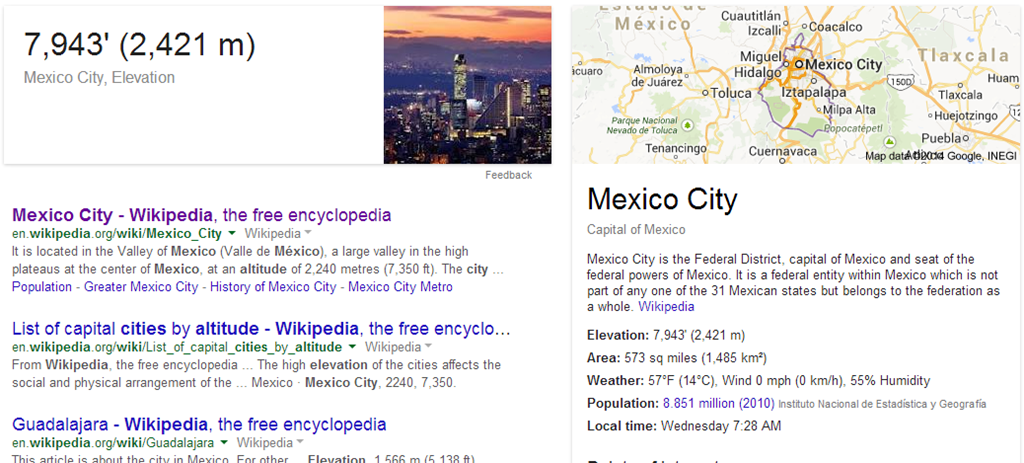This is a detailed Google search results page for "Mexico City." At the top of the page, the elevation is highlighted as 7,943 feet (2,421 meters). Accompanying this information is a picturesque image depicting the city's skyline filled with numerous buildings. Adjacent to the image is a map pinpointing Mexico City at its center, surrounded by notable locations such as Toluca and Puebla. Beneath this, the search result prominently displays the caption "Mexico City," followed by a brief description sourced from Wikipedia:

"Mexico City is the federal district, capital of Mexico, and the seat of its federal powers. It is a federal entity within Mexico, unique in that it's not part of any of the 31 Mexican states but belongs to the federation as a whole."

Further details provided include:
- Elevation: 7,943 feet (2,421 meters)
- Area: 573 square miles (1,485 square kilometers)
- Weather: 57°F (14°C), wind speed 0 mph, and humidity at 55%
- Population: 8.851 million (2010 data from Instituto Nacional de Estadística y Geografía)
- Local time: Wednesday, 7:28 AM

On the right side of the search results, the Wikipedia page for Mexico City is prominently displayed. Additional linked pages include a "List of Capital Cities by Altitude" from Wikipedia and a link to the Wikipedia page for Guadalajara.